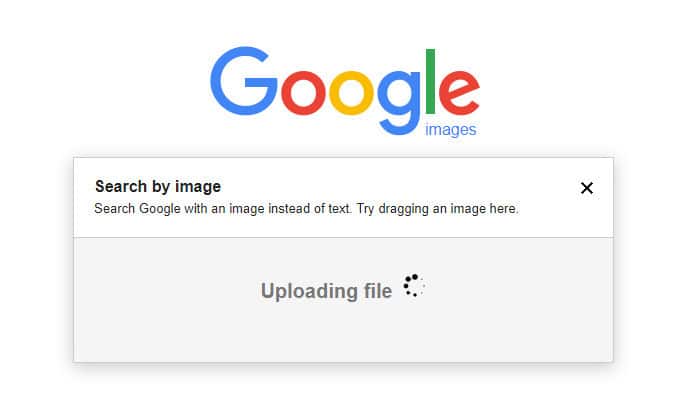Screenshot Description: A Google image search screen is depicted with a clean, white background. Centrally positioned at the top is the iconic multicolored Google logo, displayed in a sans-serif font. The first 'G' is capitalized and blue, followed by a red lowercase 'o', a yellow lowercase 'o', a blue lowercase 'g', a green lowercase 'l', and a red lowercase 'e'. Directly beneath the 'l' and 'e' of the logo is the thin, lowercase blue text reading "images."

Below the logo, a rectangular pop-up screen with sharp corners casts a light gray shadow, adding depth against the white backdrop. The pop-up is divided into two sections by a thin, medium gray line. The top section, occupying about a third of the pop-up's height, features a white background. In the top-left corner, bold black text reads "Search by image." Below this, in thinner, medium gray text, the instructions "Search Google with an image instead of text. Try dragging an image here" are displayed. A black 'X' is located at the top-right corner of this section.

The bottom section of the pop-up, taking up the remaining two-thirds of the height, has a light gray background. Centrally situated within this area is large, dark gray text stating "Uploading file." Adjacent to this text, on the right, is a circular loading animation consisting of black dots of varying sizes. The dots increase gradually in size as they form a circle, with the largest dot at the top, followed by progressively smaller dots, and then increasing in size again towards the top, creating a continuous motion effect.